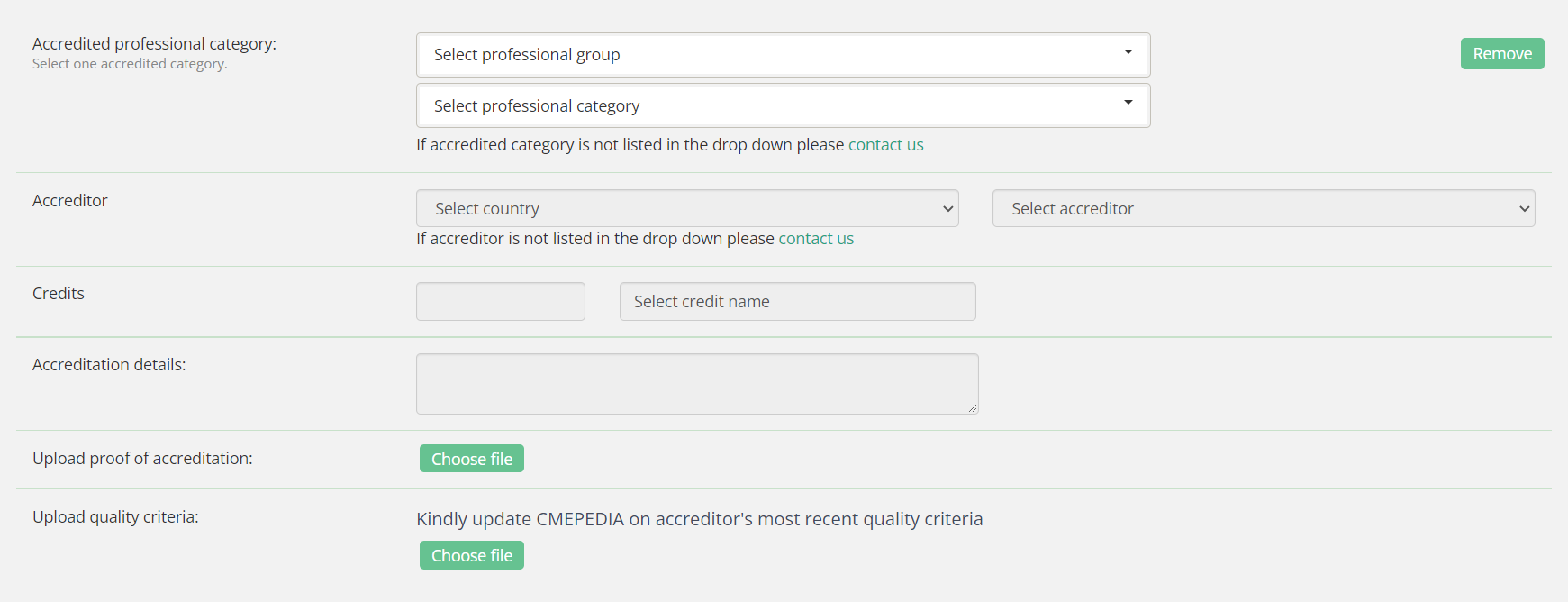In this detailed image, we see a screenshot with a light gray background and black text. In the upper left corner, there is a section titled "Accredited Professional Category." Directly beneath this title is the instruction text, "Select one accredited category." To the right of this instruction are two pull-down selection boxes. The top box is labeled "Select Professional Group," while the lower box is labeled "Select Professional Category." Below these dropdown boxes, additional instructions in black text read, "If accredited category is not listed in the drop-down, please contact us."

Moving down the image, on the left side, there is a label named "Accreditor," adjacent to which, on the right, is a pull-down box that prompts the user to "Select Country." Below this box, there is another prompt stating, "If accreditor is not listed in the drop-down, please contact us,” leading to another pull-down box labeled "Select Accreditor."

Further down, on the left side, the word "Credits" is displayed, followed by two empty fields to the right for input. Below this section, there is an option to "Upload Proof of Accreditation," accompanied by a green box with white text that says "Choose File."

The image offers a structured and comprehensive method for users to input and validate their accreditation details through a series of dropdown menus and input fields.